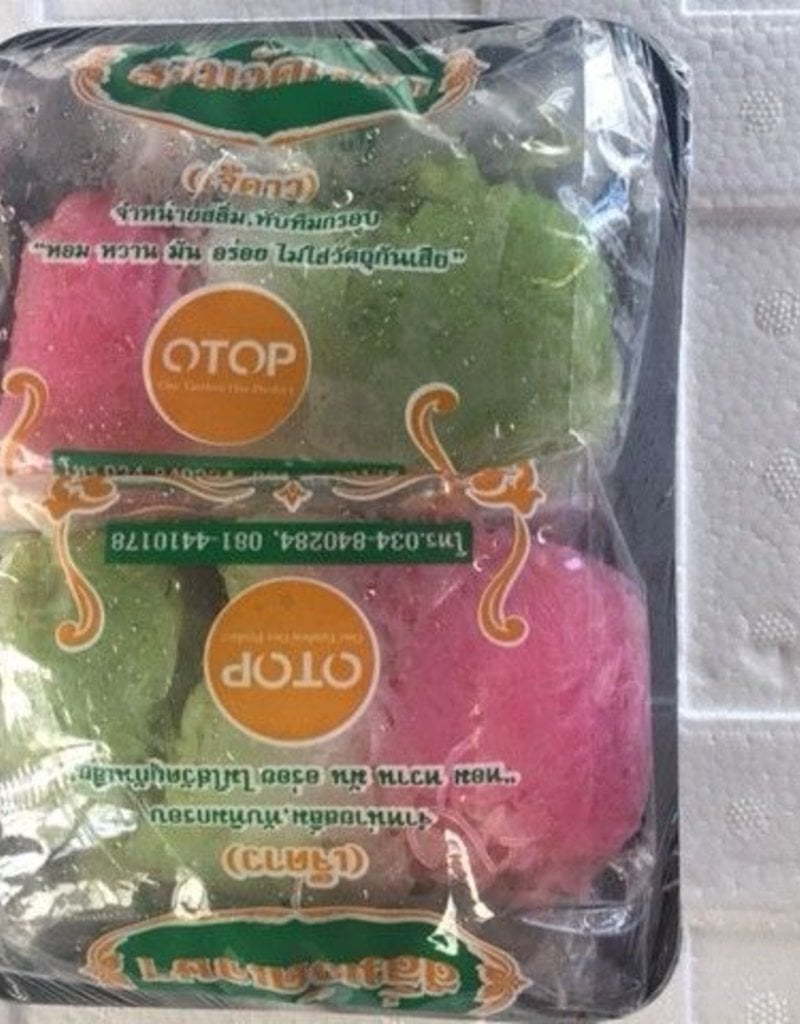The image features a display package containing gelatin-like pieces of candy, presented in a styrofoam container similar to those used for meat products. These candies, appearing wet and brightly colored in shades of pink and green, are arranged in an upside-down position in the image. The packaging displays the logo "O-T-O-P" in white font against an orange circular background. There is also another logo, a semicircular form with an orange border and green background, which contains foreign lettering. The text on the package is in a language difficult to identify. The overall composition of the image seems off-center, with the objects leaning slightly to the left, suggesting it could be set within a styrofoam cooler or shelved in a supermarket.